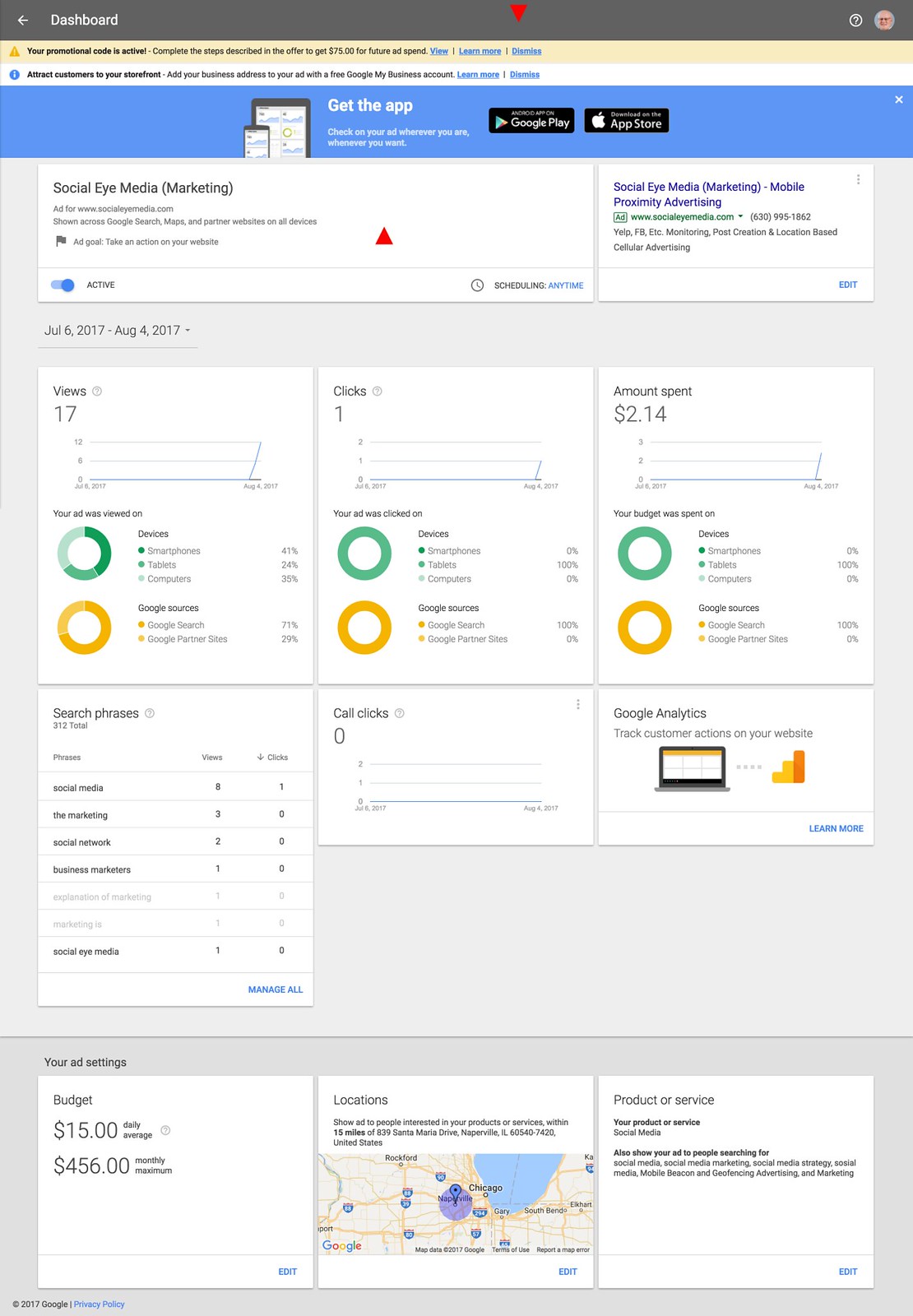The image depicts a detailed screenshot of a freelancer’s dashboard page, showcasing a comprehensive range of analytics and advertising metrics. The top banner features ads for the Google Play Store and the App Store, encouraging users to download the relevant apps.

Central to the dashboard are multiple indicators such as budget allocations, daily budget limits, and monthly spending caps. The platform provides various data points, including amounts spent, which currently display $2.14, as well as metrics for clicks, views, and call clicks. Specific terms like "search phrases," "Google Analytics," and "track customer actions on your website" are prominently mentioned, indicating the granular level of tracking available.

At the bottom, the dashboard highlights ad settings, with a budget allocation of $15 as a daily average and a monthly maximum of $4.56. The geographical focus for the ads is set to the outskirts of Chicago, tailored to reach the target audience in that location. Other elements include product or service categories and social media metrics, ensuring a holistic view of advertising performance.

Overall, the dashboard provides an extensive array of analytics, budget figures, promotional strategies, and geographical focus, all crucial for effective ad management and optimization for freelancers.